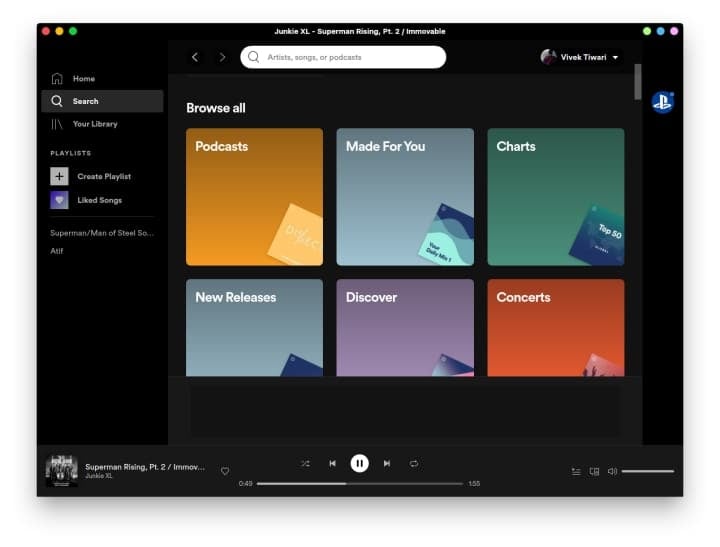This screenshot captures a music playlist and discovery application with a sleek, minimalist design featuring a black background. 

In the top left corner, three small circles in red, yellow, and green resemble a traffic light. The upper right corner showcases pale green, blue, and lavender icons, a design element seen in multiple places.

Central to the upper section, a white search bar allows users to search for artists, songs, or podcasts. Above this search bar, following the black background theme, small white text displays the current track: "Junkie XL Superman Rising Part 2, immovable."

A short vertical column on the left side lists navigation options in white text. These options include, from top to bottom:
1. Home
2. Search (currently selected)
3. Your Library
4. Playlists section with a 'Create Playlist' option marked by a plus sign icon and a 'Liked Songs' option with a heart icon

The main screen, situated to the right of this column, has a "Browse All" heading also in white text against the black backdrop. Below this heading, two rows of three square thumbnails, each featuring a small graphic, offer different categories:
- **First row (left to right):**
  - Podcasts (gold background)
  - Made For You (blue-gray background)
  - Charts (green background)
- **Second row (left to right):**
  - New Releases (pale blue background)
  - Discover (lavender background)
  - Concerts (orange background)

At the bottom of the screen, a faintly lighter shaded section delineates the playback controls, including play, pause, fast forward, and rewind buttons. The currently playing track, "Superman Rising Part 2, immovable," is shown with its album art in the lower left corner next to the playback controls.

This detailed user interface highlights the app's simplistic yet functional design, emphasizing an easy music and playlist discovery experience.